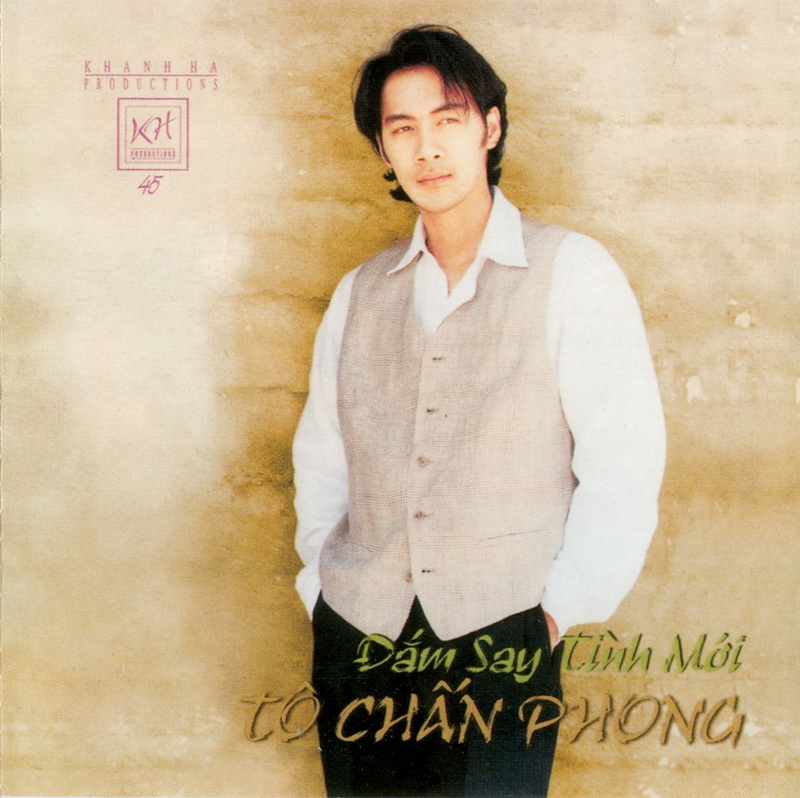A young man, who appears to be of Asian descent and likely in his mid to late twenties, is the central figure in this image. He stands against a brick wall that creates a sharp backdrop, while the areas to his left and right transition into a dreamy, bleached-out sequence. The man is dressed in a light beige or cream vest over a long-sleeved white collared shirt and black pants. His black hair is cut short, with some strands falling over his left eye, and his hands are tucked into his pockets. He gazes off to the right, just slightly out of frame.

In the upper right corner of the image, the words "KH45" are printed in purple within a circle, and just above it in purple text it reads "Kahan Productions." The lower right corner features text in an unknown language, which includes "DAM SA SAY TINH MOI" in green and "TO CHAN PHONG" in a turquoise or brownish hue. The overall atmospheric aesthetic of the image combines sharp details with dreamy, faded elements, making it an intriguing and visually compelling advertisement poster.